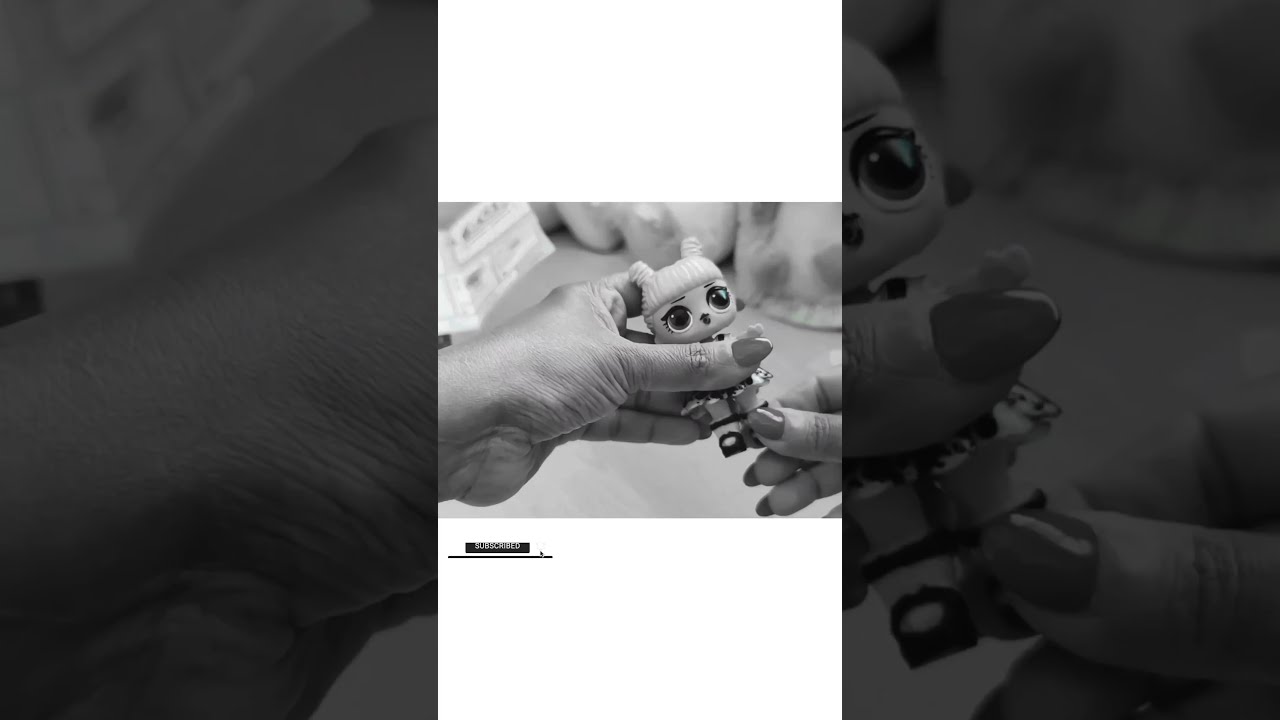The image is a black-and-white photo divided into three vertical panels. The middle panel is clear and detailed, featuring a woman's hands holding a small plastic doll. The doll, likely a female, has a large head with blonde hair styled in pigtails and big black eyes. The woman’s left hand enters from the left side, grasping the doll by the torso, while her right hand comes in from the right, holding the doll’s left foot. Her fingernails are polished red. In the background, a chest of drawers and a blanket are faintly visible. There is a small, unreadable text at the bottom that says "subscribed," suggesting a possible connection to a YouTube channel.

The adjacent left and right panels are dark and less clear, providing close-up views of the woman's hands and parts of the doll. The left panel shows her left hand and a hint of surrounding objects, potentially a dollhouse or a bureau. The right panel displays her right hand holding the doll’s foot, with other indistinct background elements like a faint blanket and some furniture visible.